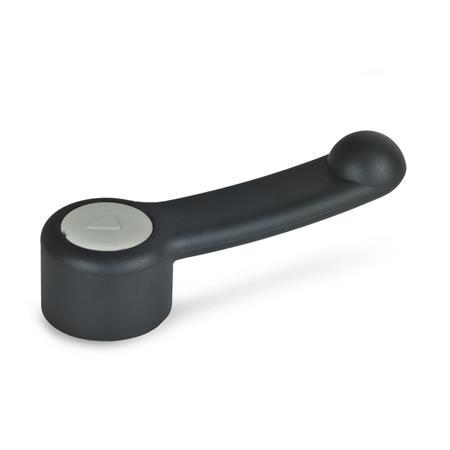The image showcases a black, plastic handle-like object positioned against a stark white background. The object consists of a cylindrical base on the left and a straight, elongated handle that extends to the right. At the far end of the handle, there is a rounded, half-ball knob, which appears to be designed for gripping. The cylindrical base features a gray circular button with a raised triangle, reminiscent of a play button, suggesting some form of directional or functional indicator. The handle, possibly with a matte black finish, seems to attach to the cylinder, possibly indicating it is used for turning or winding something. The lighting in the image comes from the right, highlighting the simple yet enigmatic design of this solitary object.